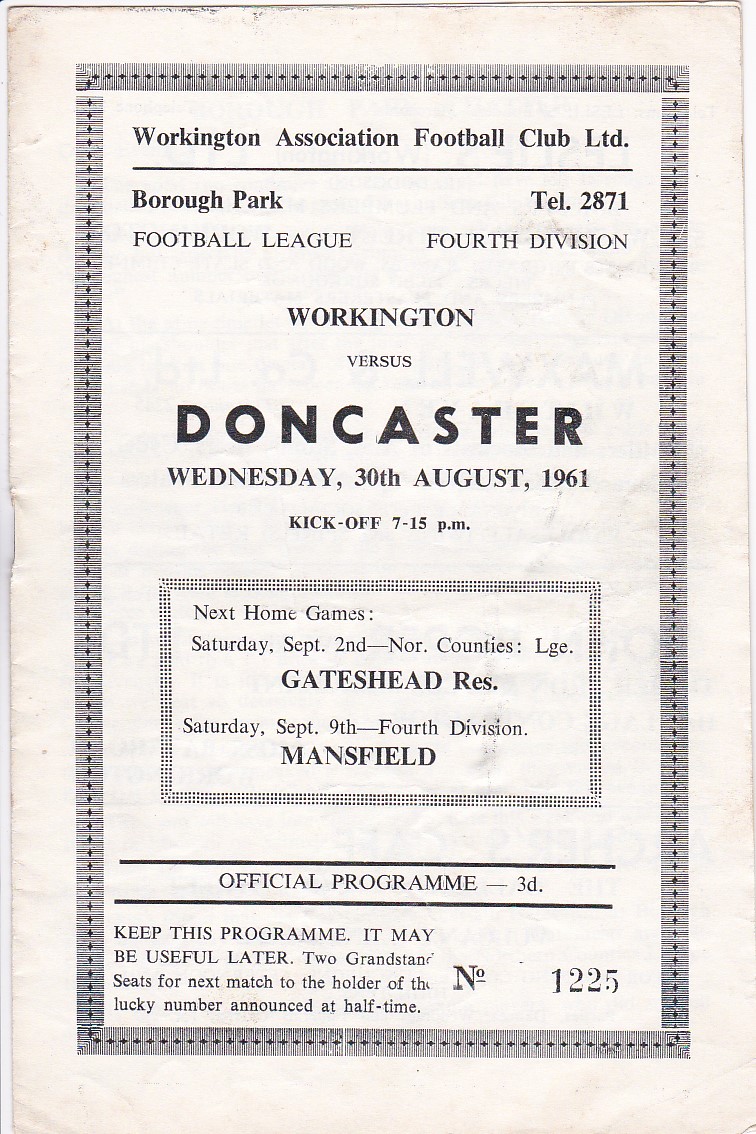The image is a portrait-oriented black-and-white print publication, specifically an inside front page of a vintage soccer program dated August 30th, 1961. The page shows signs of wear and discoloration, shifting from its original white to a grayish-brownish hue, with a staple mark on the left-hand side. A border of thin horizontal rectangles with equilateral crosses adorns the interior of the page.

At the top of the page, underlined in black, the header reads, "Workington Association Football Club Ltd." Further below, on the left, it states "Borough Park Football League" and on the right, "Tel. 2871, 4th Division." Centrally positioned, the text announces the match details: "Workington vs. Doncaster, Wednesday 30th August 1961, kickoff 7 to 7.15 pm."

A rectangle with a dotted line border encloses information about upcoming home games: "Next Home Game, Saturday September 2nd - NOR Period Counties LGE Gateshead RES, Saturday September 9th - 4th Division Mansfield." Below, bordered at the top and bottom, the text states, "Official Program - 3D."

In the lower left corner, the text advises, "Keep this program. It may be useful later." Notably, the program includes a section for a lucky draw with "Two grandstand seats for next match to the holder of number 12225," with the number 1225 stamped in the bottom right corner. The style of the page is distinctly vintage print production, capturing a piece of British football history.